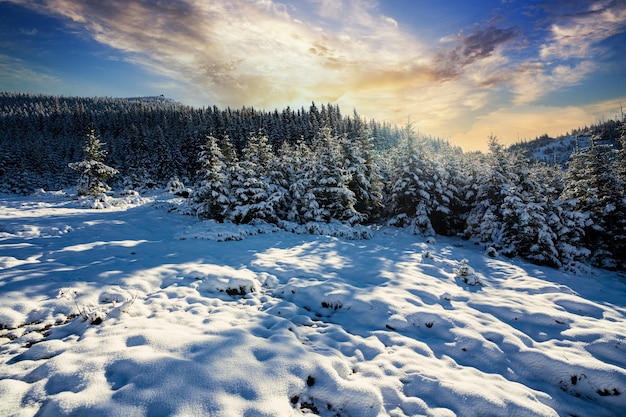This photograph captures a serene winter scene in a heavily wooded, mountainous area, possibly reminiscent of the Colorado Rockies. The foreground is blanketed with several inches of pristine, white snow with occasional patches of exposed ground, suggesting a slight thaw. Pine trees or evergreens dominate the background, their branches heavily laden with snow, creating a picturesque blend of white snow and glimpses of green needles beneath. The sky above is a bright, beautiful blue, interspersed with clouds that diffuse the sunlight, casting bluish shadows from the trees onto the snow below. It's either early morning or late evening, evidenced by the long shadows stretched across the ground, adding to the tranquil, natural beauty of this winter landscape. The image, devoid of any text, exudes a crisp, cold atmosphere, making one almost feel the chill of the winter air.